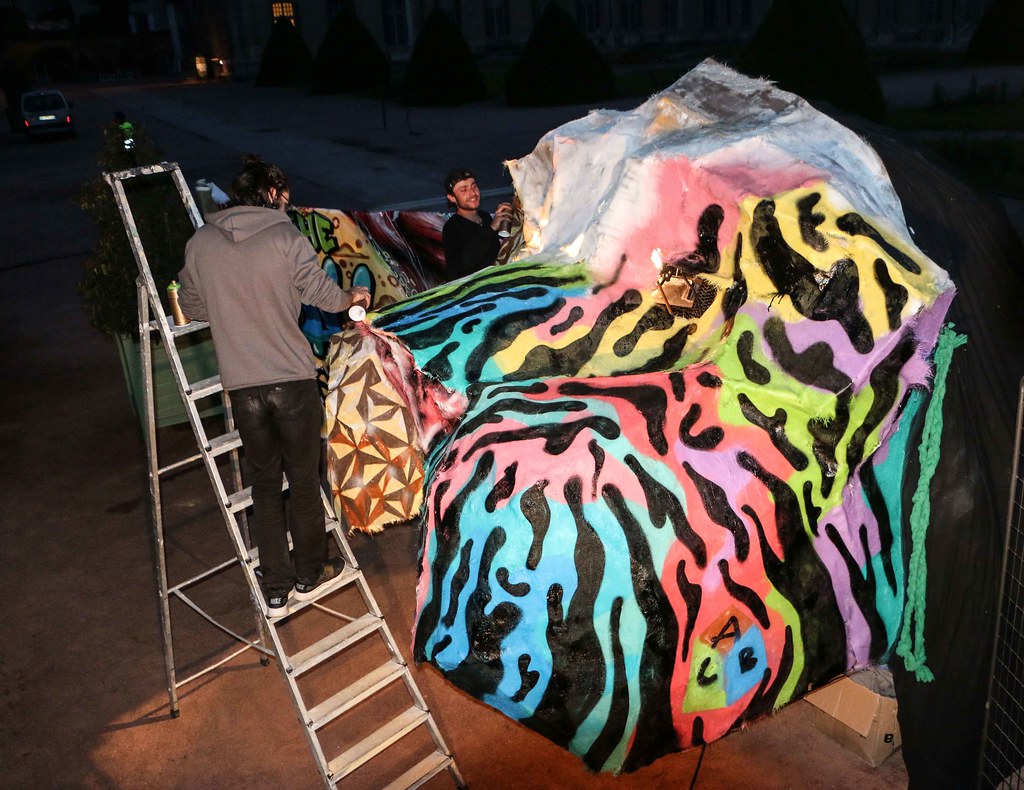The photograph captures a nighttime scene where two individuals are engaged in painting a very large rock, or potentially a makeshift structure or tarp, in a vibrant, modern graffiti style reminiscent of Keith Haring's work. The painting features a multitude of vivid, 80s-esque colors including blue, red, green, yellow, purple, and pink, with black squiggly designs overlaying these hues. 

On the left side of the image, one of the artists, dressed in black pants and a gray sweatshirt, stands on a ladder while holding a golden spray can in their right hand. Their back is to the camera, revealing short black hair. On the right, another individual, wearing a backwards black hat and a black shirt, smiles slightly while holding a black spray can. This person's facial features suggest European descent.

In the foreground, a cube with "ABC" on its faces can be discerned. The background of the image reveals a dark, nighttime setting with a dimly lit street, a parked car, and a partially illuminated house with a single window glowing in the distance. Additional lighting appears to be set up to illuminate the work area, ensuring the artists can see their canvas clearly despite the night.